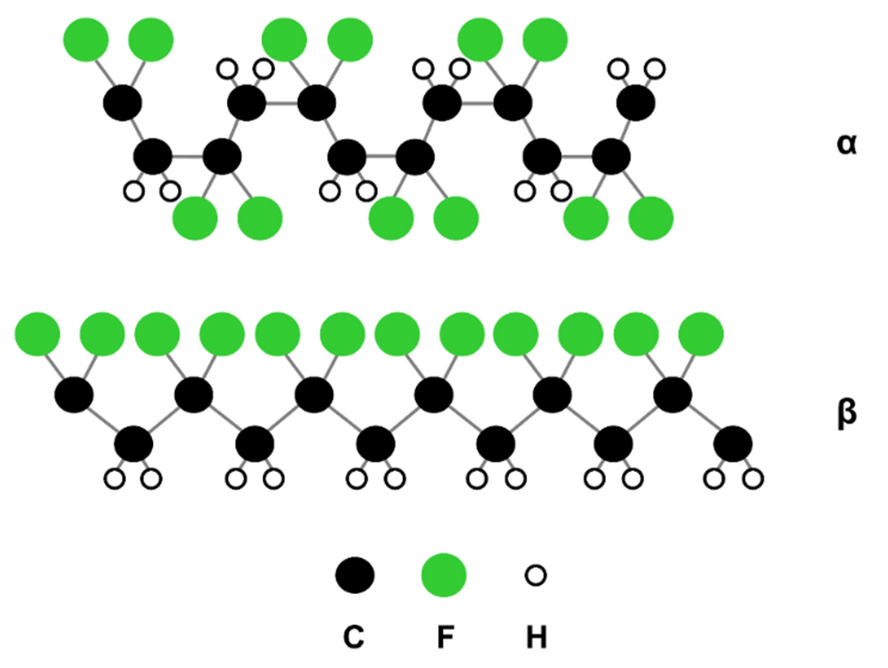The image illustrates two detailed diagrams labeled A and B against a white background, suggesting a textbook-style depiction of molecular compounds. Each diagram consists of various colored circles, representing different atoms, connected by lines indicating chemical bonds. Diagram A showcases an intricate network with approximately 30 circles arranged in four to five rows and ten columns. The circles are colored green, black, or white, with green circles (labeled F) being the largest, black circles (labeled C) slightly smaller, and white circles (labeled H) the smallest. In Diagram A, green circles appear at the top and bottom, black circles are centrally located, and white circles are positioned in between. Diagram B is slightly wider, featuring a linear arrangement where green circles are at the top, followed by black circles in the middle, and white circles at the bottom. Although the diagrams appear complex, no key is provided to precisely identify what each labeled element represents.